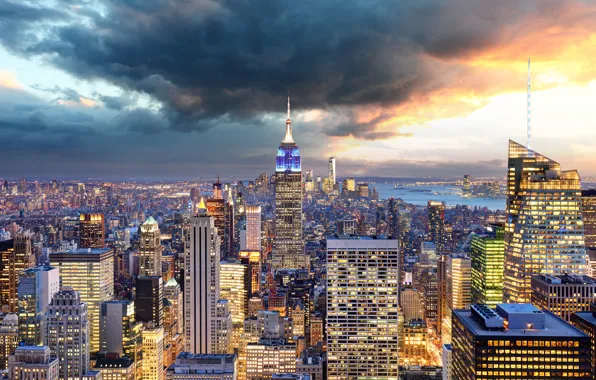The image is a highly detailed color photograph, likely of New York City, capturing a dramatic twilight scene. Dominated by a bustling cityscape, the photograph prominently features numerous skyscrapers and buildings, each illuminated against the gathering darkness. Notably, the Empire State Building stands tall in the center, cloaked in blue lights at its peak, possibly accompanied by the sharp spire of the Chrysler Building adding to the iconic skyline.

The sky above is an arresting mix of elements: to the right, the sun is setting, casting a fiery red and golden-orange glow that lights up part of the sky and the buildings below. The breathtaking illumination contrasts sharply with the dark, looming storm clouds dominating the center and left of the image, creating a sense of impending weather turmoil. Underneath these dramatic clouds, the city lights shimmer, undeterred by the gathering gloom.

On the right-hand side of the photo, a river—possibly the Hudson—can be seen weaving through the expanse of urban structures, with lights from a neighboring borough like Hoboken twinkling along its banks. The scene overall captures the dynamic energy and atmospheric tension of a city on the brink of a storm at twilight.